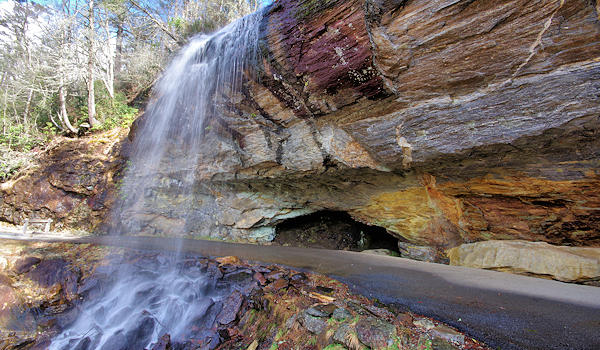This image depicts an artificial waterfall cascading down a multi-layered rocky cliff face, set in a natural outdoor environment. The waterfall, positioned towards the left side of the picture, flows over a rock formation which displays a range of colors from beige at the bottom, through darker shades in the middle, to red at the top. The rock layers resemble shale or limestone and include a small, shallow cave at the base. Surrounding the waterfall, the cliff is bordered by a walking trail that allows viewers to experience the scene up close. In the background, several bare, deciduous trees suggest a season either in fall, early spring, or winter, set against a bright blue sky dotted with fluffy white clouds. The overall mood is peaceful, accentuated by the medium flow of the waterfall and the striking contrast of the colorful rock formations.